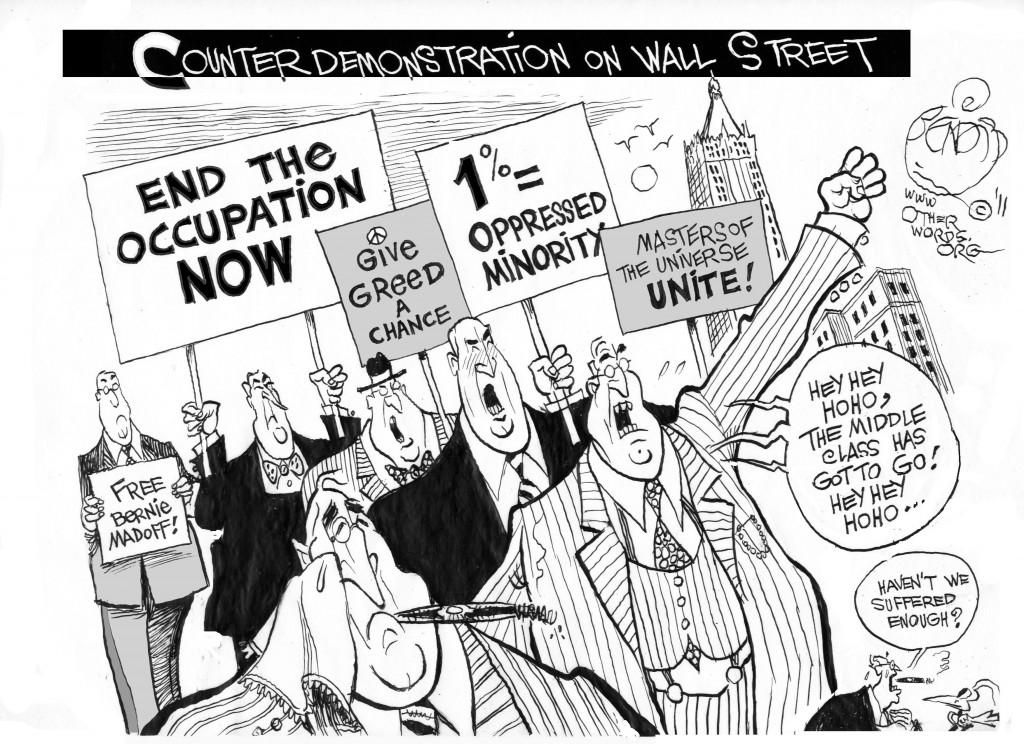This detailed black-and-white political cartoon, presented in landscape orientation, vividly captures a satirical scene highlighting the affluent's mock protest against the middle class. Dominating the top of the image, a horizontal black bar features the handwritten phrase "Counter Demonstration on Wall Street" in white letters. Below this, a group of old, white, overweight businessmen clad in fancy three-piece suits and ties, some smoking cigars, hold various protest signs. The signs read: "End the Occupation Now," "Give Greed a Chance," "1% = Oppressed Minority," "Masters of the Universe Unite," and "Free Bernie Madoff." The businessmen are portrayed chanting "Hey, hey, ho, ho, the middle class has got to go," with one prominently at the foreground leading the chorus. Another businessman, depicted crying and wiping away tears, holds a sign that says "Haven't we suffered enough?" The scene, likely set in New York City, is underscored by a tall skyscraper, birds flying, and a sun in the background. In the upper right corner, the artist’s signature and a copyright symbol are visible, along with the text "otherworld.org," contributing to the cartoon's framing.